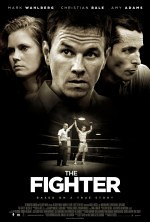This is a black and white poster for the movie "The Fighter," featuring a gradient effect that fades to black around the edges. The title, "The Fighter," is prominently displayed at the bottom in large white text, accompanied by the movie credits below. Above the title, there’s an evocative still image of a victorious boxer in a ring, with a referee raising the boxer's hand in triumph. The central area of the poster displays three faces: on the left is a white woman with light brown or possibly ginger hair, identified as Amy Adams; in the middle is Mark Wahlberg with short brown hair, and on the right is a profile shot of Christian Bale with very short dark hair. All three actors are featured in their roles from the movie. The background is predominantly dark, adding to the dramatic effect of the poster.